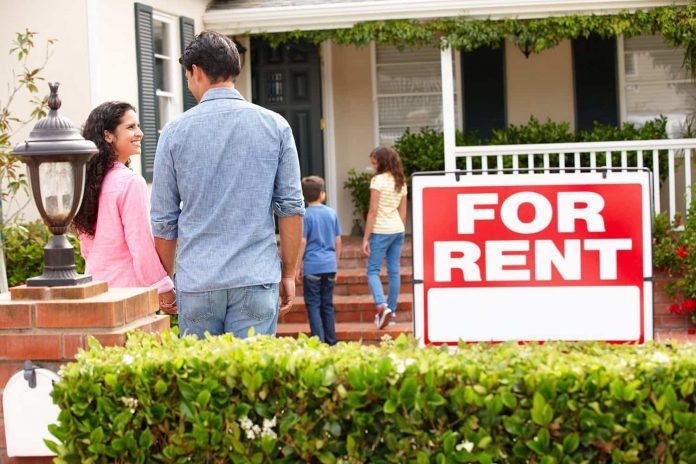The image shows a charming, white, two-story house available for rent, prominently featuring a red "For Rent" sign with white lettering in the foreground. The sign is positioned above a well-trimmed, square-shaped bush. To the left of the bush stands a mailbox embedded in red bricks, accompanied by a copper lamppost. A couple, seemingly delighted, is prominently visible to the left, with the woman dressed in a pink shirt and the man in a blue collared shirt and blue jeans, walking hand in hand towards the house. Just ahead of them, two children, a boy in a blue shirt and light blue jeans, and a girl in a yellow striped shirt, are playfully ascending the red brick steps that lead to the porch. The inviting porch, adorned with a white railing, sports green plants, and the house itself features a blue door and blue shutters. The scene captures a warm, welcoming atmosphere as the family approaches their new rental home.